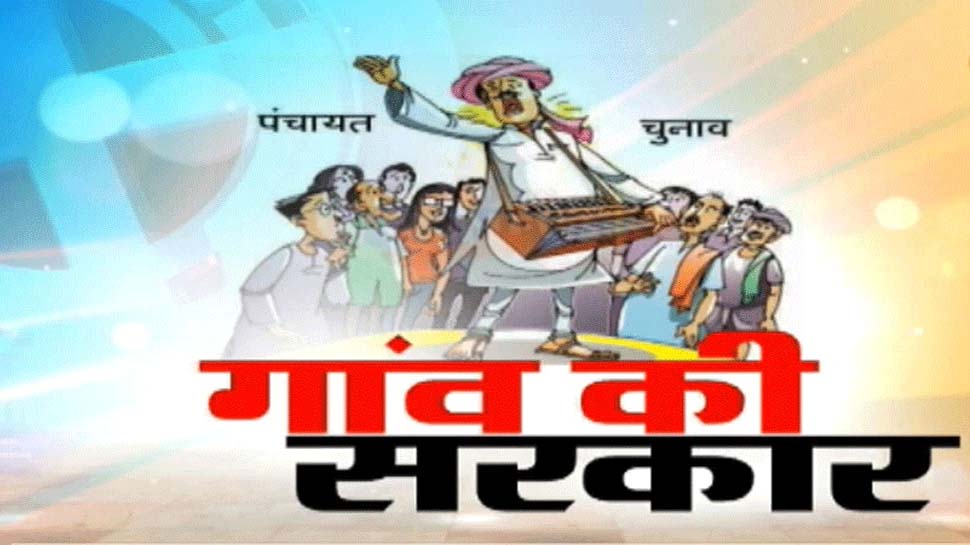The image appears to be an advertisement featuring a computer-generated blend of animation and surreal graphics. At the center is a cartoon depiction of a man, possibly of Middle Eastern or Indian descent, dressed in a white linen outfit with a red turban. He's performing by playing a squeeze box or keyboard, his right arm outstretched as if singing or shouting. Behind him, a large crowd of people, depicted in a cartoon style, are in awe, watching his performance. Notably, a young girl in an orange shirt and blue jeans stands among the crowd, emphasizing the diversity of the group. The background features a blue, somewhat transparent circle with lines and subdued rays of light emanating from behind the crowd. At the bottom, there is bold text in a mix of red and black, written in Arabic or a similar language, serving as the title or headline of the advertisement.